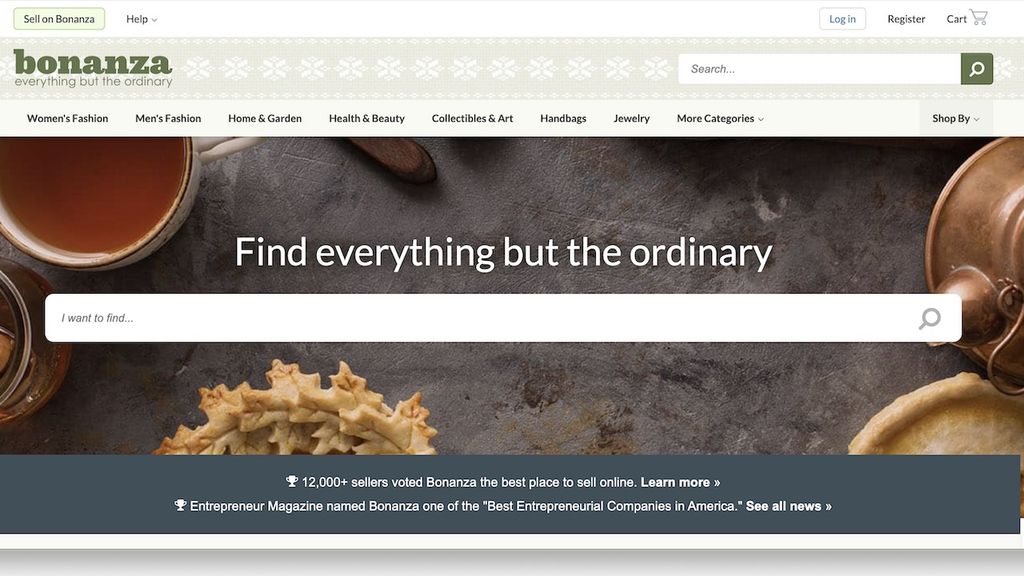This screenshot captures the homepage of the Bonanza website, showcasing various UI elements and features. At the top, a white navigation bar is present, highlighted by a light yellow-green box. Within this box, the black text reads "Sell on Bonanza" and beside it, a "Help" button with a dropdown arrow appears. On the right side, there is a white box with the text "Log In," followed by "Register," and then a cart icon with the word "Cart."

Below the top navigation, a white-green strip featuring subtle snowflake icons stretches across the page. Centered within this strip, the green text spells out "Bonanza: Everything but the ordinary." Nestled beneath this slogan is a white search box with an adjacent green button displaying a white magnifying glass icon, labeled "Search."

Descend further and you encounter a series of black submenu links including "Women's Fashion," "Men's Fashion," "Home and Garden," "Health and Beauty," "Collectibles and Art," "Handbags," "Jewelry," and "More Categories," which has an arrow indicating a dropdown menu. Adjacent to these submenus, a light green button labeled "Shop By" with a small arrow is visible.

An image dominates the subsequent section, depicting a gray table surface adorned with various items: dough cut into leaf shapes, a copper kettle, a fragment of another pie, a cup of orange tea, and a jar possibly containing cinnamon. Below this image, a white search box appears again with the phrase "Find everything but the ordinary" and a gray magnifying glass icon. Inside the search box, the placeholder text reads "I want to find..."

The lower portion of the page features a navy blue section with white text centered around two trophy icons. The text states, "12,000+ sellers voted Bonanza the best place to sell online. Learn more," and further notes, "Entrepreneur Magazine named Bonanza one of the best entrepreneurial companies in America."